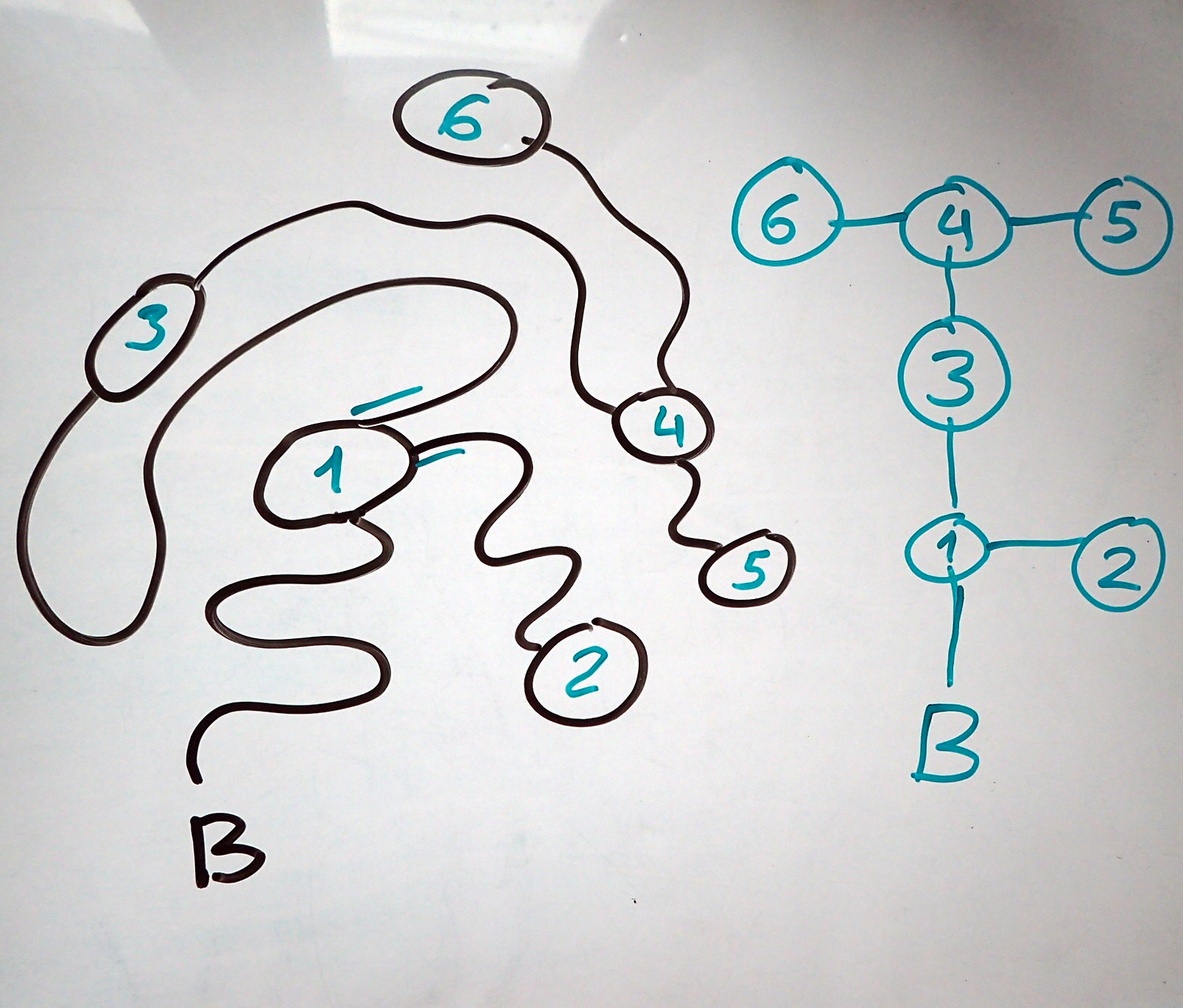The image captures a whiteboard that reflects fluorescent lighting, causing parts of the surface to appear in varying shades of black. Two fluorescent lights are visibly reflected in the top left corner. The whiteboard is marked with both dark teal and black markers, creating an intricate diagram.

To the right, there are several teal numbers within black circles, connected by various lines. Specifically, dark teal markings include a "B" and a series of lines connecting numbers enclosed in circles. For example:
- A line connects a teal "1" with a black circle to a teal "2" with a black circle, situated to its right.
- Above this, a line connects teal "3" with a black circle below to teal "4" with a black circle above, intersecting lines to both the left and right.
- To the left, a teal "6" with a black circle links to the connecting structure, while a teal "5" with a black circle is connected on the right.
- At the bottom left, there’s another "B" and a sequence of switchback loops and partial loops.

Below these, an additional series of details requires description:
- A teal "1" with a black circle, featuring a switchback line leading down to a teal "2" with a black circle, and another incomplete teal line trailing off.
- At the top, a black line leads to a teal "3" with a black circle around it, followed by a large loop to the right.
- From this "3," a teal marking at the start of the circle connects to more squiggly lines.
- A squiggly line extends to teal "4" with a black circle, linking further with a black squiggly line to teal "5" with a black circle. 
- The teal "4" also connects via a long squiggly line to teal "6" with a black circle above.

Overall, the whiteboard is filled with a complex network of interconnected numbers and shapes, creating a detailed and engaging visual.